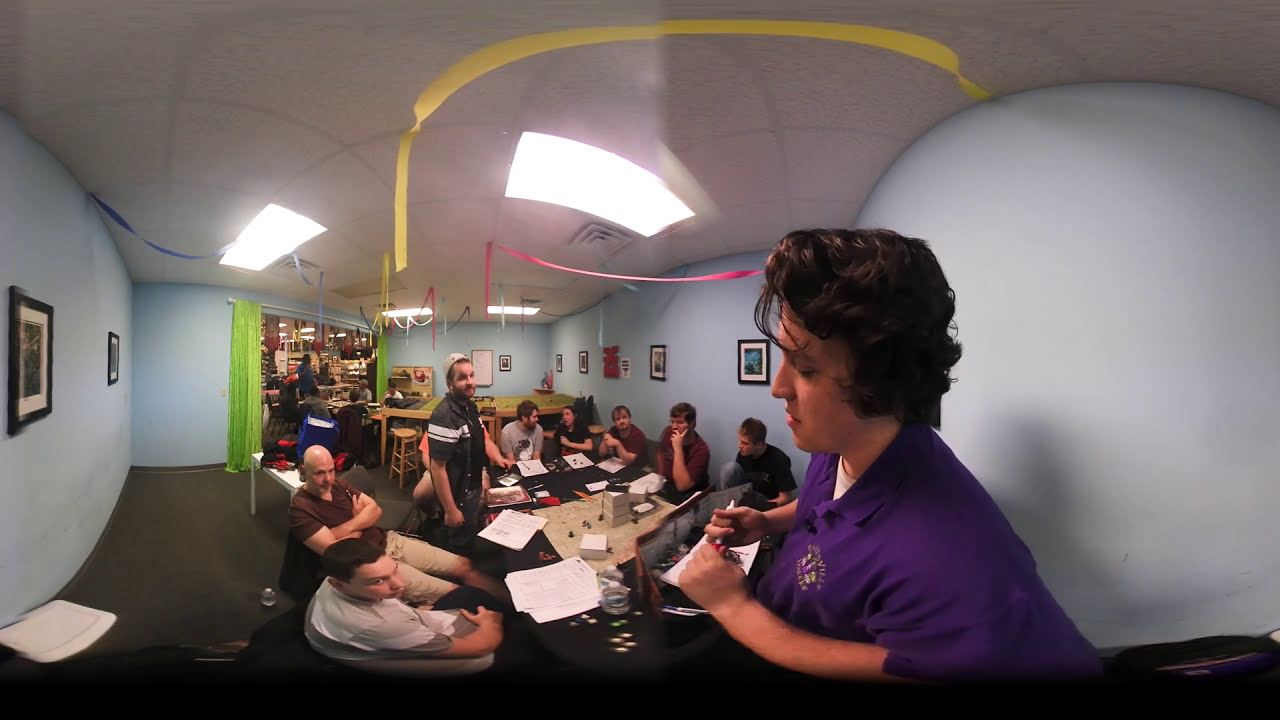The panoramic 360-degree image showcases the interior of a brightly lit room with light blue walls resembling various shades such as bird shag, birdshell, and birds egg blue. The ceiling is an off-white drop panel type with a gray metal framework, adorned with yellow, blue, and pink streamers that add a festive touch. On the back wall, a large open doorway framed by green curtains provides a focal point.

In the immediate foreground, a woman with short brown hair is seen in a short-sleeved purple polo shirt, seemingly initiating or leading the gathering. Surrounding her is a conference table where nine to twelve individuals, mostly Caucasian, are seated and engaged in conversation, some holding menus. Notable figures include a Caucasian man with dark, curly hair also in a purple polo shirt, appearing to be looking at a menu or writing, and another man standing by the table in a black shirt with white stripes. A bald man in a brown polo shirt and tan shorts, and another man in a gray t-shirt with dark hair are also visible. The room gives off a dynamic atmosphere, possibly indicating a meeting or a classroom-like environment, with everyone focusing on the woman at the forefront. The photo's distortion and warping, especially around the ceiling, suggest it was taken with a 360-degree or VR camera, enhancing the immersive experience of the scene.